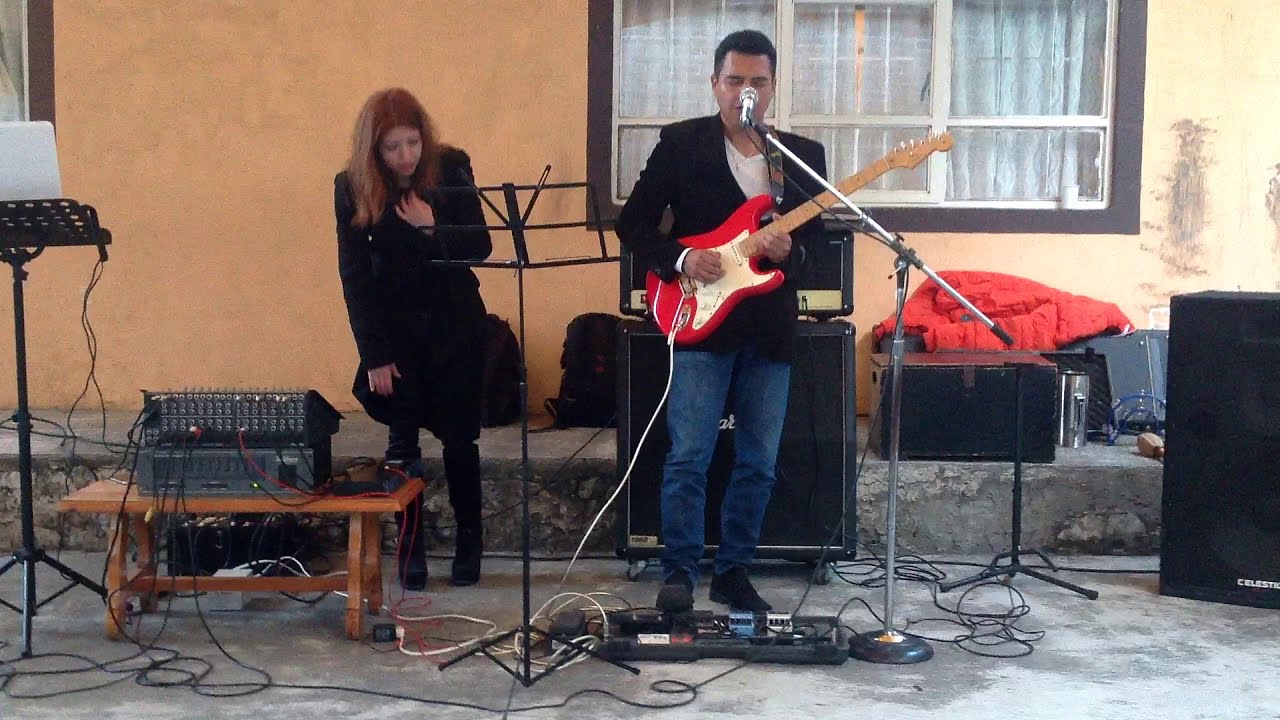In this detailed outdoor image, a man stands in the center, in front of a house with a window in the background, playing a red and beige guitar plugged into a large black amplifier speaker situated behind him to his right. Dressed in a black jacket over a white t-shirt, blue jeans, and black boots, the man is captured with his eyes closed and mouth slightly open, suggesting he is singing into the microphone set in front of him. To his left stands a woman with long brown hair, clad in a black jacket, intently looking down at the pedals on the concrete slab beneath them, which could be a patio or sidewalk area. Scattered around are various pieces of musical equipment, including another microphone on a stand, a music stand without sheet music, and numerous wires connected to a large electronic musical device. A red jacket is draped over some additional speakers to the man’s right. The overall scene suggests they might be practicing for a performance or engaging in an impromptu jam session, with the setting appearing somewhat run-down, perhaps indicating a garage or makeshift practice space.